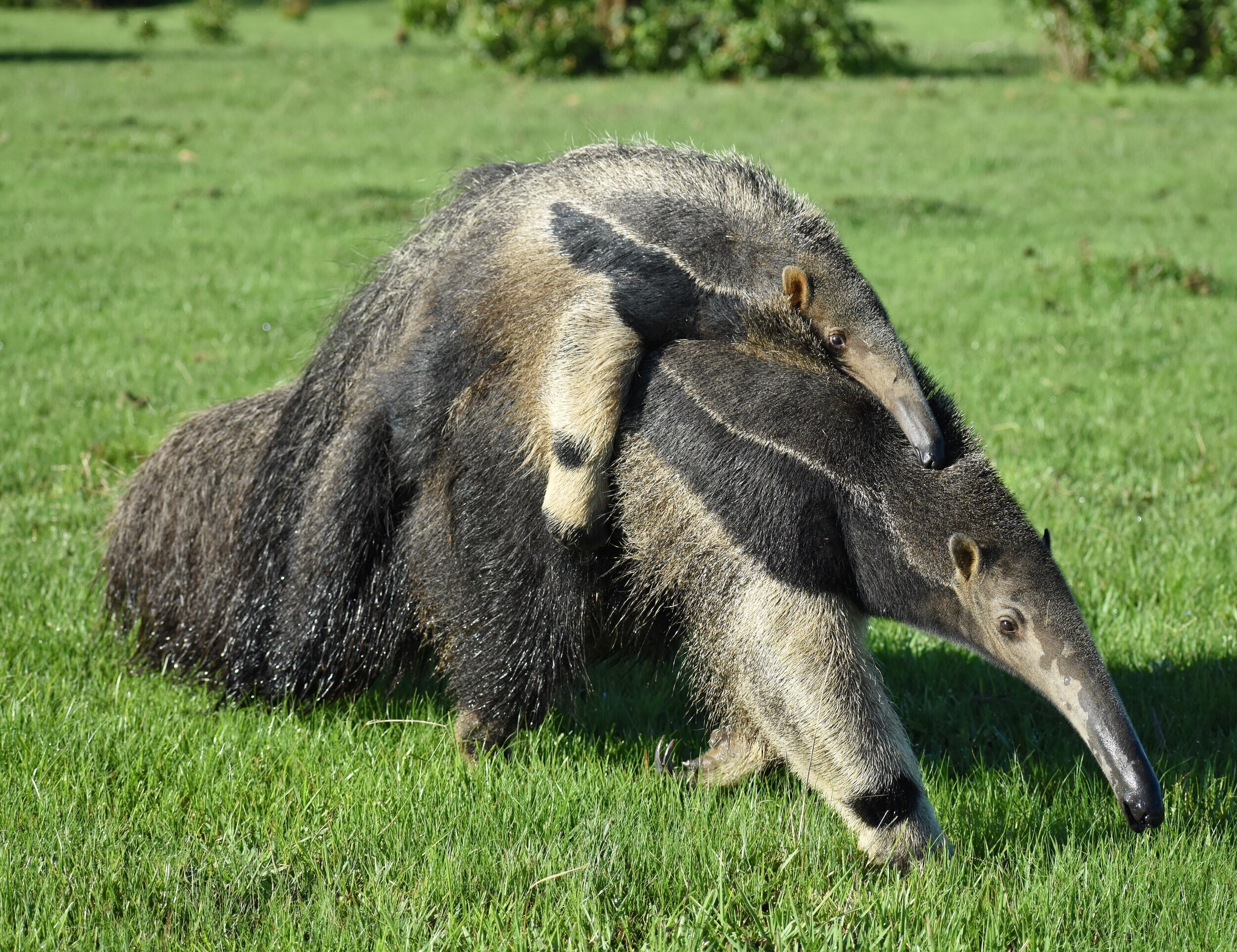This professional landscape photograph captures a rare and striking scene of two anteaters in a grassy pasture with some distant shrubbery. Pointing towards the right, a larger adult anteater is walking while carrying a smaller juvenile on its back, which rests atop the adult's body. Both animals have remarkably long snouts and small, beady eyes, with ears that are dark and pointed. Their coats are a mix of dark black and brown fur, with their legs blending into a creamy color and highlighted by patches of light, blondish tan fur. Their tails are notably bushy, adding to the overall texture of their flat, furry appearance. The vivid green grasses and smattering of trees create a bright and natural backdrop for this extraordinary and endearing depiction of the anteaters in their natural environment.